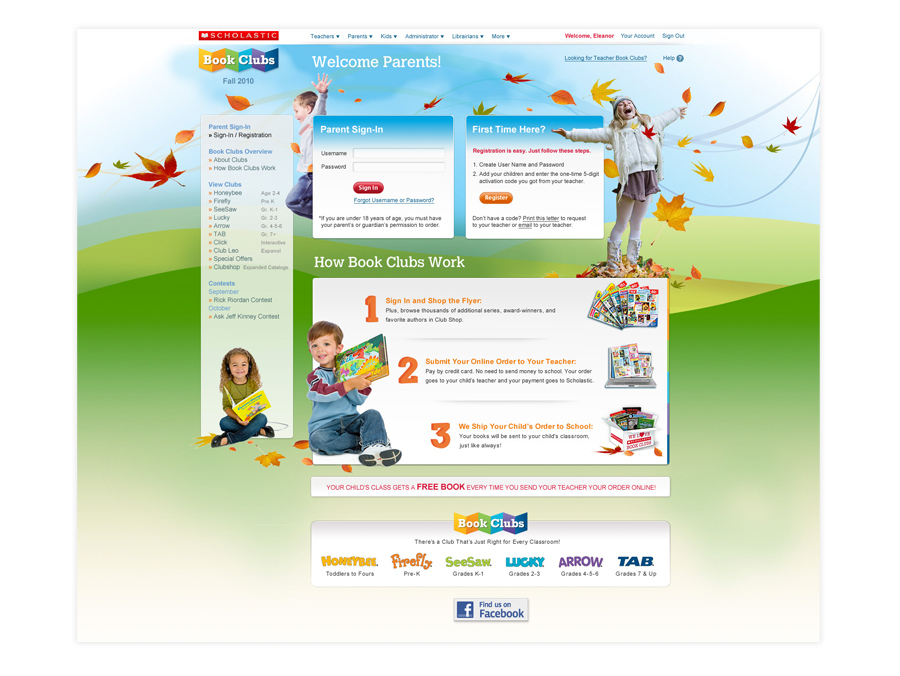The image features a prominently displayed Scholastic banner on the top left, with the word "Scholastic" in white letters against a red background. The navigation bar includes drop-down menus labeled "Teachers," "Parents," "Kids," "Administrators," "Librarians," and "More." On the far right, the red text reads "Welcome eLearner," next to links for "Your Account" and "Sign Out." Just below this, a heading reads "Book Clubs Fall 2010" with a "Welcome Parents" message. To its right, there is a link that says "Looking for Teacher Book Clubs?" followed by a "Help" link.

The main section of the webpage is dedicated to a parent sign-in area, requesting a Username and Password with options for "Forgot Username" and "Forgot Password." There is a note advising that children under 18 must have parental or guardian permission to order. For first-time visitors, instructions explain that registration is simple: Step one is creating a username and password, and step two involves adding children and entering a five-digit activation code provided by their teacher. There are options to print a request letter for the code or email the teacher.

The website outlines how the book clubs work: Step one is signing in and shopping the flyers; step two is submitting the online order to the teacher; and step three is shipping the child’s order to their school. On the left side, information is provided about various book clubs, their contents, and monthly themes. Additionally, there's an overview of book clubs and a parent sign-in space.

At the bottom of the page, a note highlights that a child’s class receives a free book with every online order a parent sends to the teacher. There are also social media links to "Find Us on Facebook." The book clubs cater to different age groups: "Honeybees" for toddlers to flowers, "Firefly" for Pre-K, "Seesaw" for grades K-1, "Lucky" for grades 2-3, "Arrow" for grades 4-6, and "Tab" for grades 7 and up.